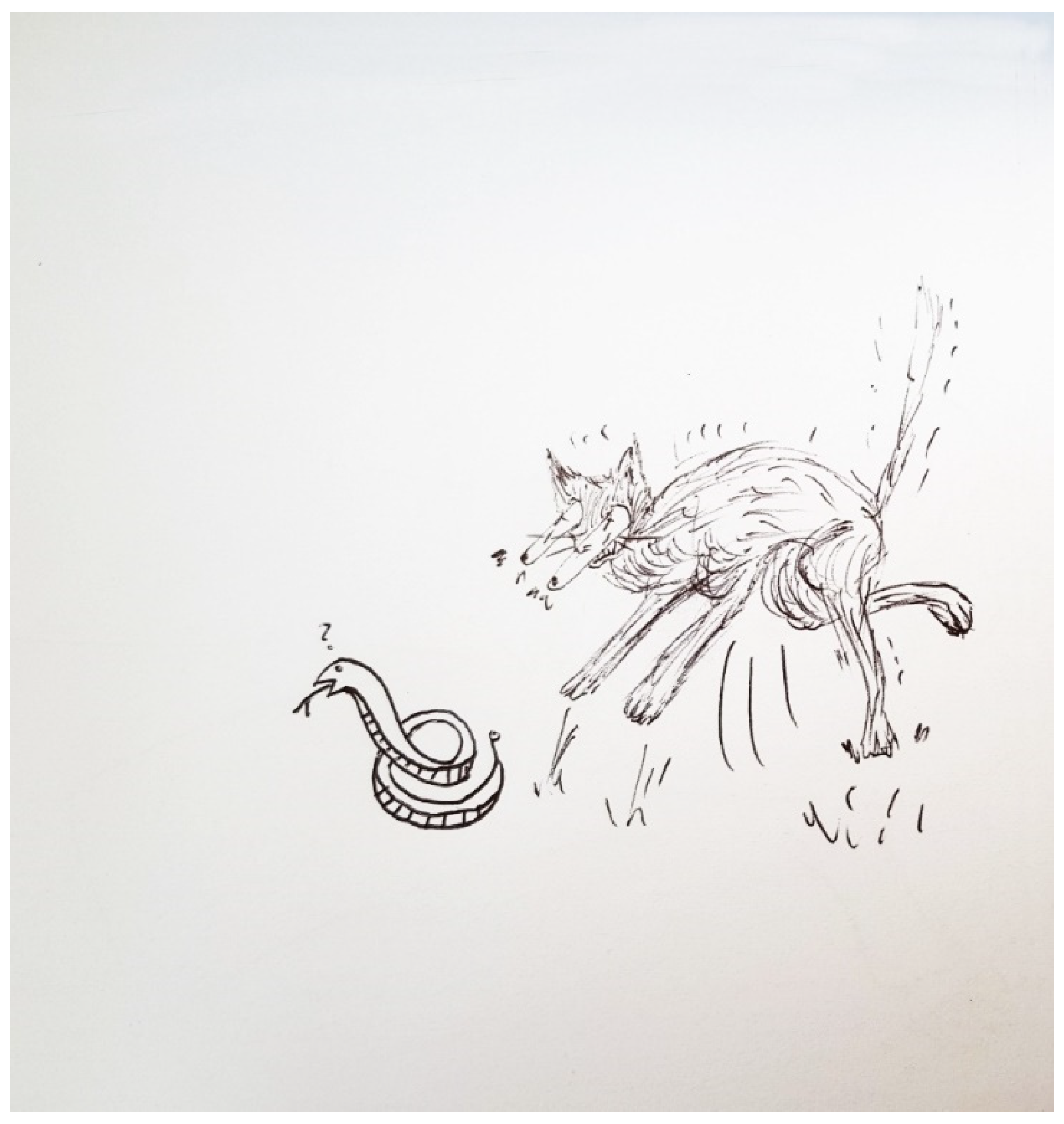The image features a detailed black-and-white pencil sketch on a white background, depicting a dynamic interaction between a cartoonish cat and a coiled snake. The snake, positioned centrally towards the bottom of the paper, is intricately drawn with solid, consistent lines and has its head lifted with a forked tongue sticking out, forming an upside-down Y. Above the snake, there is a question mark suggesting confusion or curiosity. The snake's body coils under itself, with darker shadowing lines visible beneath its white top body.

Behind the snake, more faintly sketched, is a cat with exaggerated features, notably its bulging eyes that suggest surprise or intent focus on the snake. The cat, drawn lightly but with expressive lines, appears to be in mid-leap from the right side of the image, oriented left towards the snake. Its front legs are extended outward while its rear right leg is kicked up off the ground, indicating movement. The cat's tail is held straight, and there are lines around it that imply action or motion, as if it is pouncing or running through grass.

Overall, the contrast between the solidly drawn snake and the lightly sketched, animated cat adds a sense of depth and lively interaction to the image.